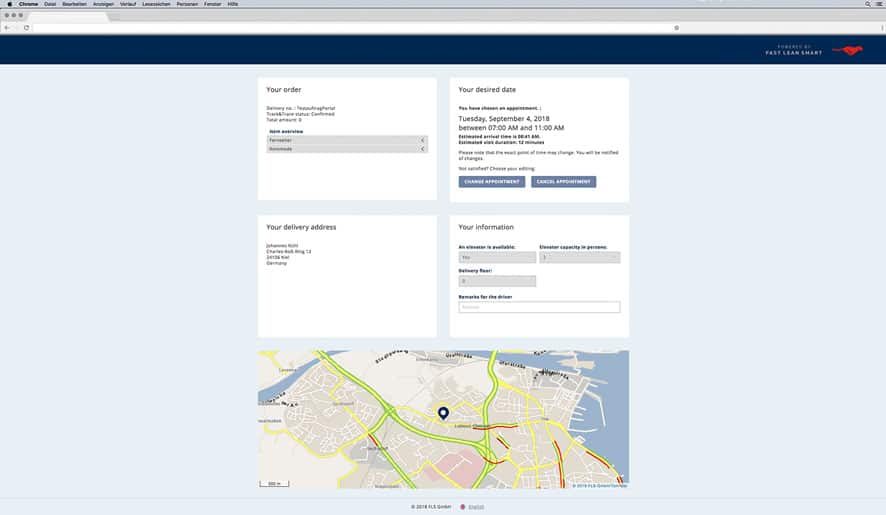The image displays a computer screen with a specific tab open, seemingly designed for digital teaching or instructional purposes. The tab is titled "Your Order," prominently displayed in a white rectangle at the top. Below the title, the screen is divided into four distinct sections; two at the top and two at the bottom.

In the first section, "Your Order," there are text details and a rectangle listing two items. Adjacent to this, on the right side, the section labeled "Your Desired Date" specifies the delivery date and time: Tuesday, September 4th, 2018, between 7:00 a.m. and 11:00 a.m. Underneath this, two clickable buttons are visible: one labeled "Cancel Appointment" and the other one partially obscured and unreadable.

The second section, located below the first, is titled "Your Delivery Address," containing a text box with the specified delivery address.

In the third section, "Your Information," towards the bottom right, there are three gray input boxes and one additional box at the bottom likely meant for user information input.

Finally, the fourth section features a map at the very bottom of the screen with a single pin marking a specific location. This structured layout on the screen aims to provide a clear and orderly presentation of the order and delivery information, suitable for instructional purposes.